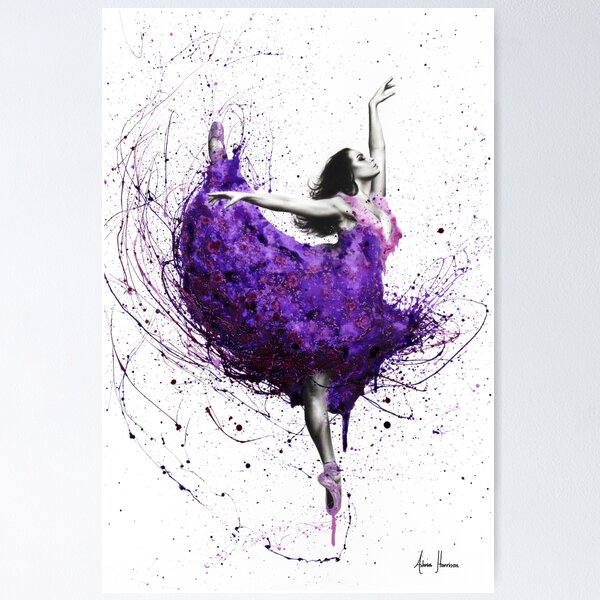In this portrait-oriented painting, set against a light gray wall with a white background, we see a mesmerizing sketch of a ballerina, seemingly floating without a visible floor. The ballerina is captured standing tiptoe on her right toe, her left leg high and arching backward gracefully behind her. She has long, dark hair flowing behind her, and wears a sleeveless, deep purple dress with splashes of lighter purple and hints of pink flowers. Her left arm is elegantly raised above her head towards the right corner of the picture, with her right arm extended horizontally to the left. The artwork radiates energy through dynamic brush strokes of purple and black lines that create swirling patterns around the dress, adding a sense of movement. Tiny black dots and drips of paint further enhance this effect. In the bottom right corner, barely legible, is the artist's signature, possibly reading "Alameda Harrington".